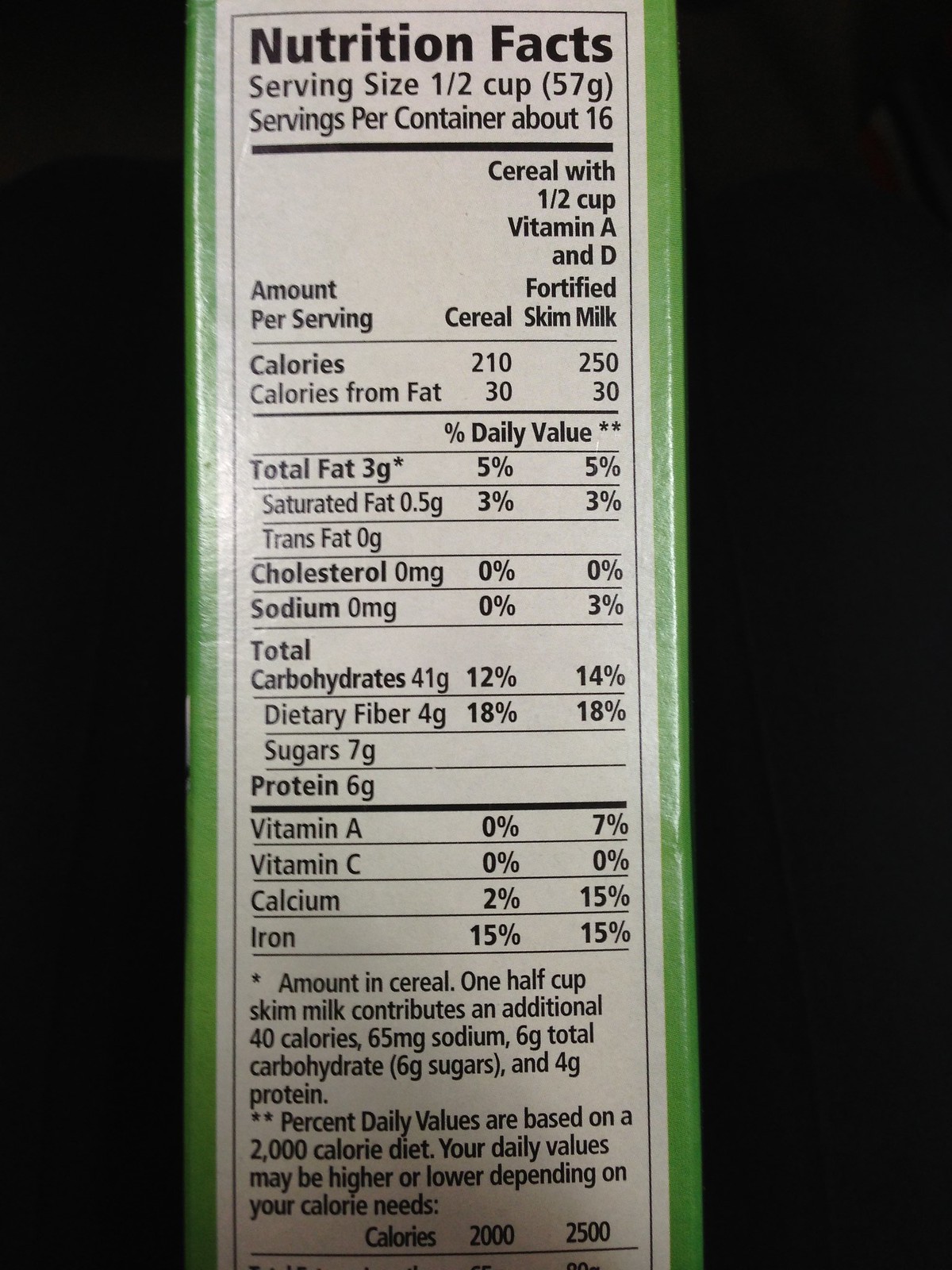Image Description: 

The image showcases a detailed nutritional information label with black bars framing the left and right edges. At the top, the title "Nutrition Facts" is prominently displayed. Beneath it is the serving size, listed as "Half-Cup (57 grams)" with approximately 16 servings per container.

There is a dividing line, and to the right side, there is specific nutritional information for "Cereal" and "Primary Vitamin B," referencing "Half-Cup" servings. The details are divided between cereal alone and cereal with skim milk.

Caloric content is shown as 210 calories for cereal alone and 250 calories with skim milk. Calories from fat are consistent at 30 calories in both cases. For total fat, the label reads 3 grams (5% of the daily value), with saturated fat at 0.5 grams (3% DV) and no trans fats. Cholesterol and sodium are both marked at 0 milligrams.

Total carbohydrates are listed as 41 grams, constituting 12% of the daily value for cereal alone and 40% with skim milk. Notably, sugars account for 7 grams and protein for 6 grams. 

Vitamin A and Vitamin C both contribute 0% of the daily value for cereal alone, increasing to 7% with skim milk. Calcium makes up 2% of the daily value without milk and 5% with it. Iron is notable at 50%, consistent with or without milk.

Additional notes specify that a serving of 1.5 cups of cereal with skim milk adds approximately 40 calories and varies in contributions such as sodium and total fats. The daily values are based on a 2,000 calorie diet, although individual requirements may differ. A comparative chart is provided for calorie intakes of 2,000 and 2,500 calories.

This detailed chart helps in understanding the nutritional contribution of eating this cereal either alone or with skim milk, aiding consumers in making informed dietary choices.